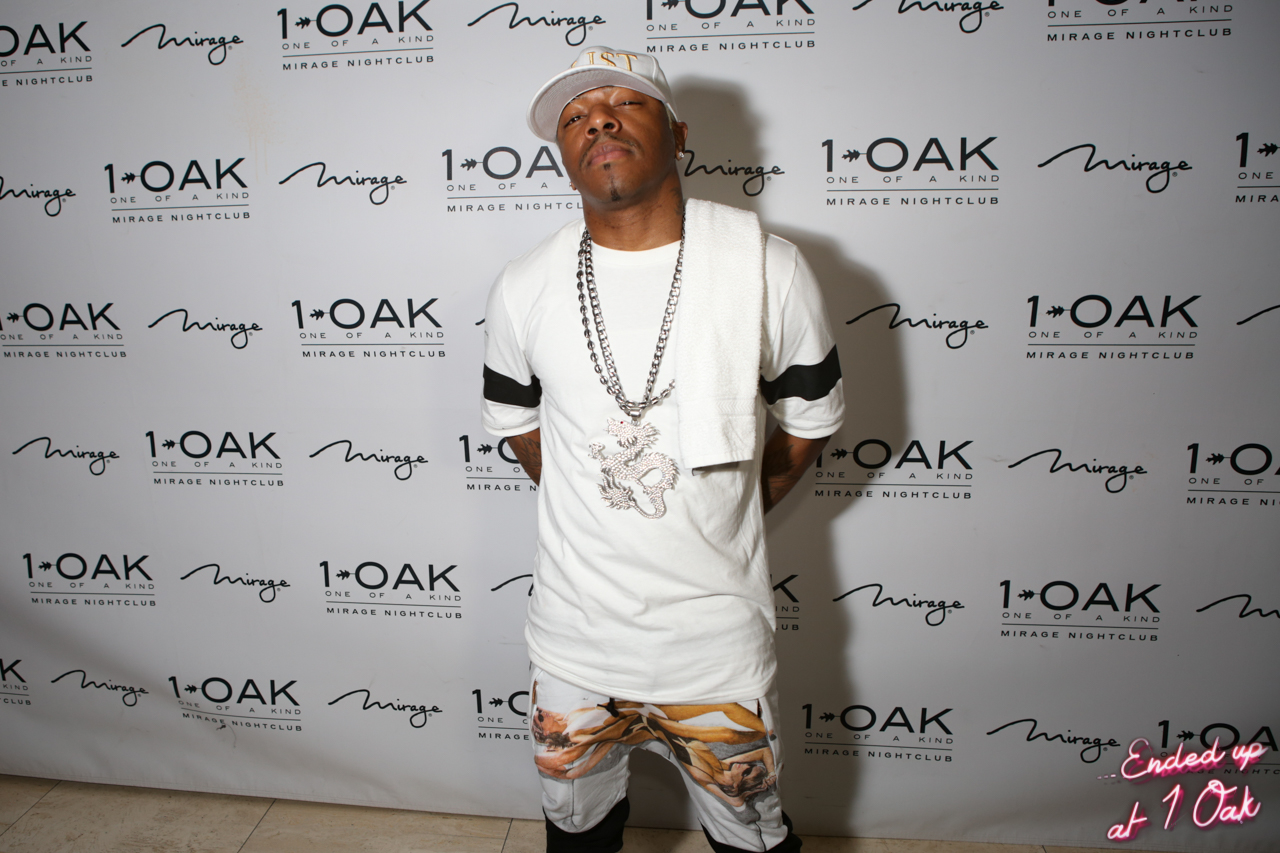In this indoor photo, an African-American man, possibly a celebrity or rapper, poses confidently against a backdrop promoting the Mirage Nightclub's One Oak event. He's dressed in a white, short-sleeve t-shirt with distinctive black stripes around the arms and a prominent dragon symbol in the center. Adorning his neck is a striking gold chain featuring a dragon pendant. He wears a white flat-brim cap with gold writing and has a white towel draped over his left shoulder. His white shorts have a logo, seemingly depicting women in bathing suits, adding a unique detail to his outfit. The man's accessories include a diamond earring and visible tattoos on his arms, which he holds behind his back. The backdrop behind him repetitively displays the text "One Oak Mirage," along with the tagline "one of a kind Mirage nightclub," with a watermark reading "ended up at One Oak" in the bottom right corner.